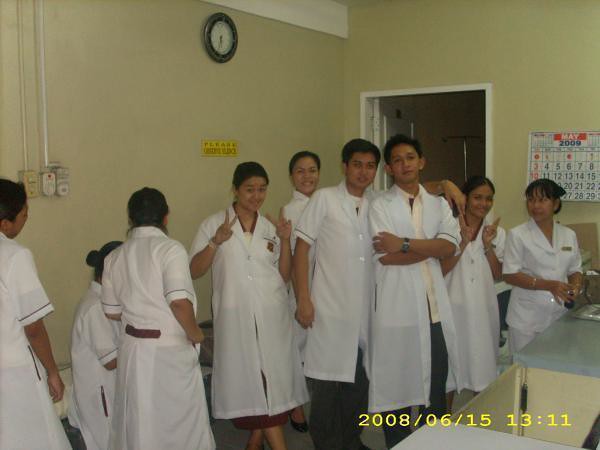The photograph, taken on June 15, 2008 at 13:11, captures a group of Asian medical students or professionals in a facility with beige walls. They are predominantly dressed in long white lab coats, though some wear nursing uniforms or street clothes underneath. The mood is mixed, with a few individuals smiling and engaging with the camera, including a female who's making a peace sign, while others focus elsewhere. A clock on the wall to the right reads 6:30, and a calendar on the back wall oddly displays May 2009. A countertop adorned with various items runs in front of the group. Metal equipment with pipes is also visible. Notably, one male in the center has a watch on, and another female is gesturing with gang signs, adding a casual and light-hearted touch to the professional setting.